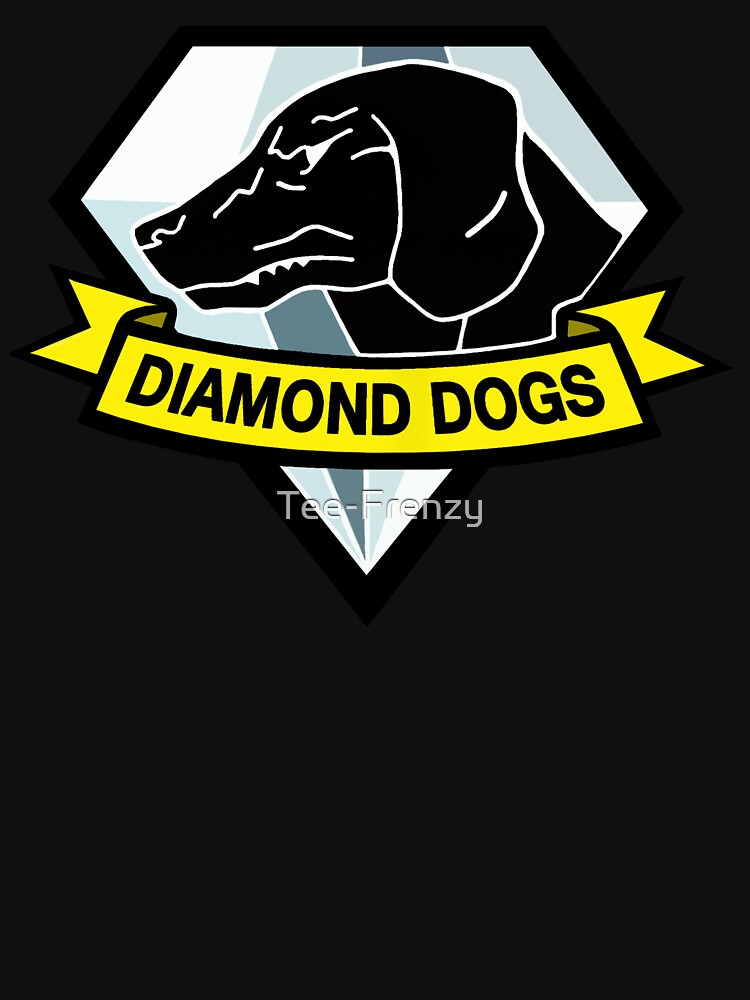The image showcases a detailed logo design reminiscent of the TV show Ted Lasso. Positioned against a blackish-gray background, the logo features a diamond with a gradient of white to light blue, transitioning to dark blue and back again to light blue. At the center of the diamond, a menacing black dog with white outlines and features, growls as it faces the viewer, almost like a silhouette. Below the dog's profile, a yellow banner with bold black text reads "Diamond Dogs." At the bottom tip of the diamond, a faint watermark says "T. Frenzy." This emblematic design, with its strong contrasts and vivid details, suggests a logo for a company or team represented by T. Frenzy.